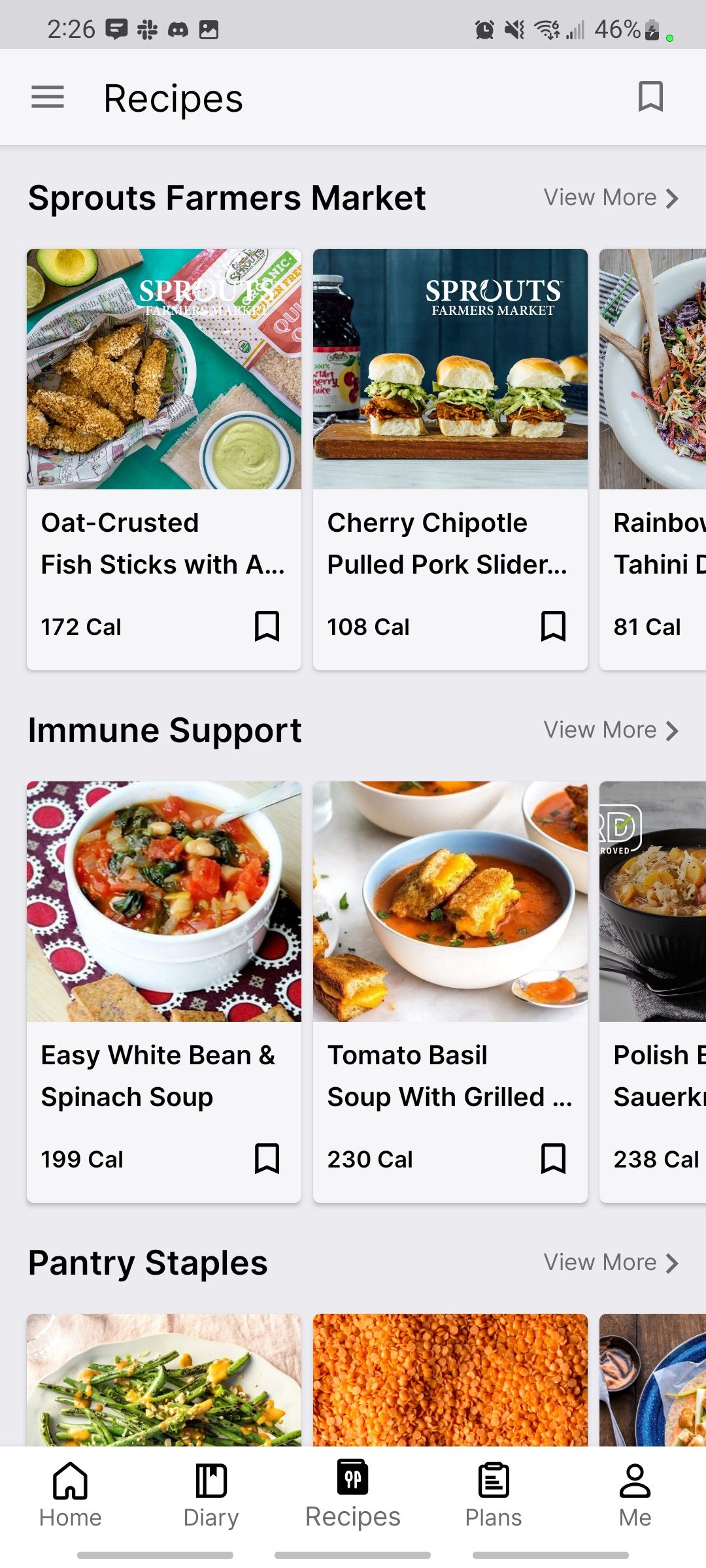This image showcases a website viewed on a mobile phone. At the very top, there's a gray border with black print displaying "226" alongside various icons - a game controller, a chat symbol, an alarm clock, a speaker with a dashed line for volume, Wi-Fi signal, cell phone signal, the text "46%", a battery icon, and a green dot. 

Below this, the website's main content begins. The background is white, featuring a prominently displayed "Recipes" heading. Underneath the white section, a darker gray background bears the text "Sprouts Farmers Market" with a "View more" link accompanied by a right-pointing arrow.

Lower down, different food images are displayed, along with calorie information:
1. "Oat Crusted Fish Sticks" with 172 calories.
2. "Cherry Chipotle Pulled Pork Spider" with 198 calories.
3. Part of the next image is cut off.
4. "Immune Support Easy White Bean and Spinach Soup" with 199 calories.
5. "Tomato Basil Soup with Grilled Cheese" with 230 calories.

Further down, two additional images are cut off, and beneath them, it reads "Pantry Staples", followed by the "View more" text. The rest of the content is not visible.